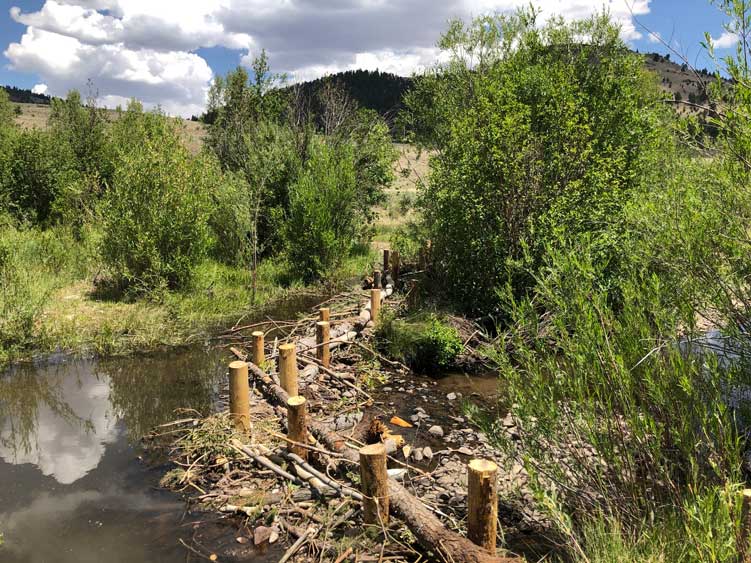In this outdoor nature scene, a wooden structure resembling a dilapidated bridge or old fence stretches diagonally from the bottom right to the top left of the image, then shifts direction and extends horizontally into the distance. The structure is made of weathered wooden poles and cross planks, with some vertical and horizontal logs still visible despite its messy and degraded state. To the left of this wooden path, there is a muddy pool of water, and to the right, a small creek or stream flows parallel to the path, weaving through the dense surrounding vegetation of grass, plants, bushes, and trees. The ground around the water is strewn with rocks, branches, and other natural debris. Overhead, the sky is mostly cloudy with occasional patches of blue, and behind the scene, gently rolling hills covered in greenery add depth to the landscape.